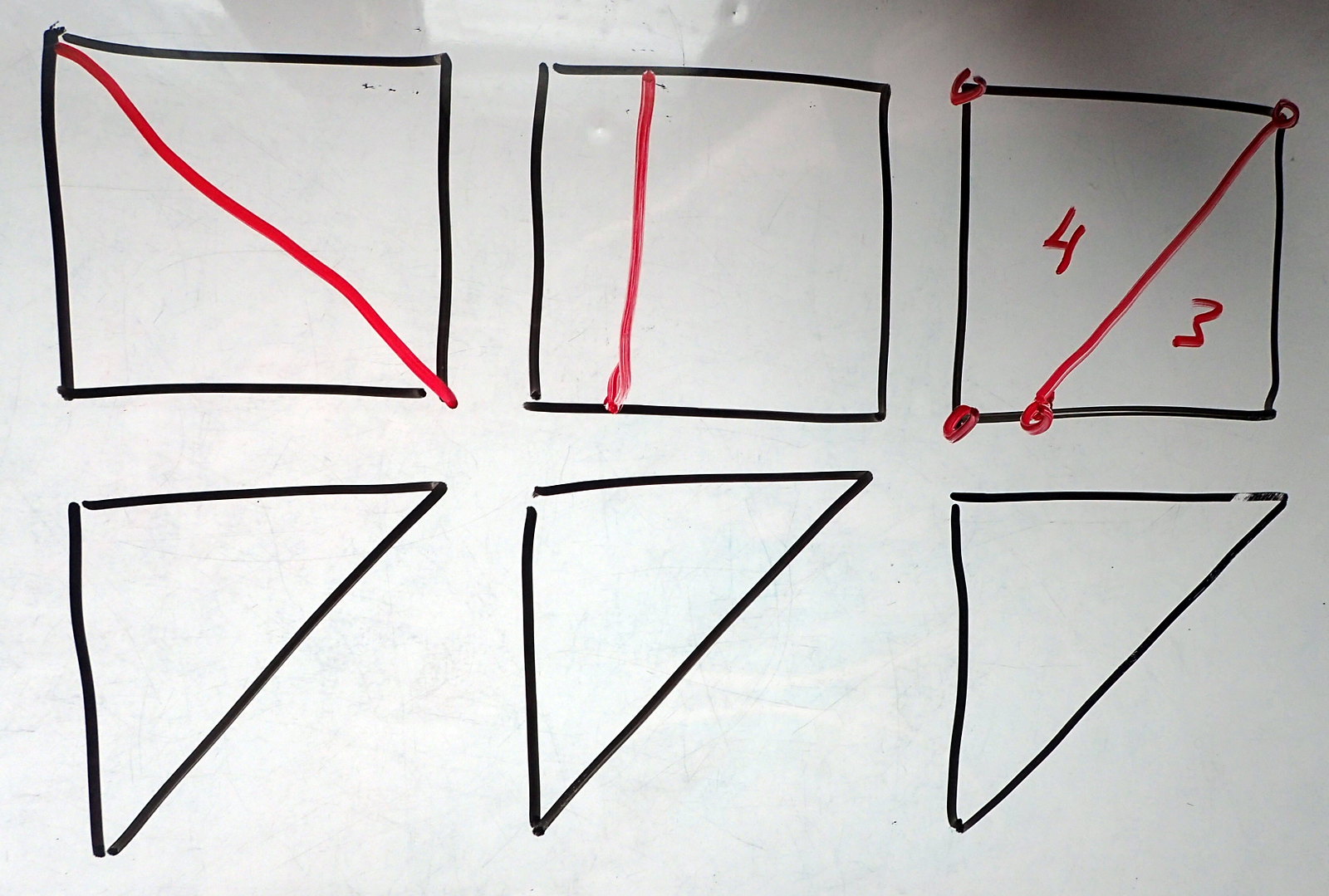The image depicts a slightly wrinkled piece of paper set against a white background. In the upper left corner of the paper, there is a black square drawn with a marker, featuring a red diagonal line stretching from the upper left corner to the lower right corner. To the right of this square, there is another black square, which has a vertical line running from the top to the bottom. Further to the right, a third black square is present, marked by a diagonal line going from the upper right corner to the lower left corner. Additionally, this square's lower left, upper left, and upper right corners are encircled in red. The numbers "4" and "3" are written in separate halves of this square. Along the bottom portion of the paper, there are three black triangles aligned diagonally, with their points oriented toward the upper left corner of the image. A light source is situated behind the camera, causing a noticeable glare in the upper middle section of the image, adding a reflective quality to the scene.